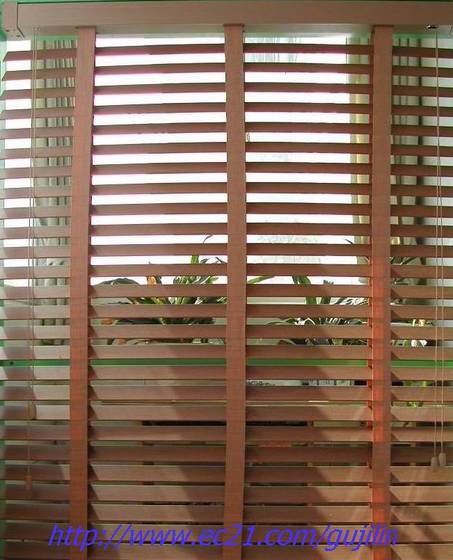The image depicts a set of horizontally arranged wooden blinds, brownish in color with a hint of red, possibly made from cedar. The blinds are partially open and facing downward, allowing a glimpse into another room. Both the left and right sides of the blinds have tan-colored drawstring cords hanging down. The threading used in the blinds is also tan, with the block holding them in place matching the brown color of the blinds. Through the slats of the blinds, the scene reveals a bright, sunlit area, suggesting it is daytime outside. In the other room, visible through the blinds, are green plants with long, lanceate leaves, which might be dracaena plants, situated on a table or desk. No curtains are visible, but there are green drapes that add to the lush, verdant look of the other room. Spanning the bottom of the image in purple text is the website address, "http://www.ec21.com/G-U-J-I-L-L-N."